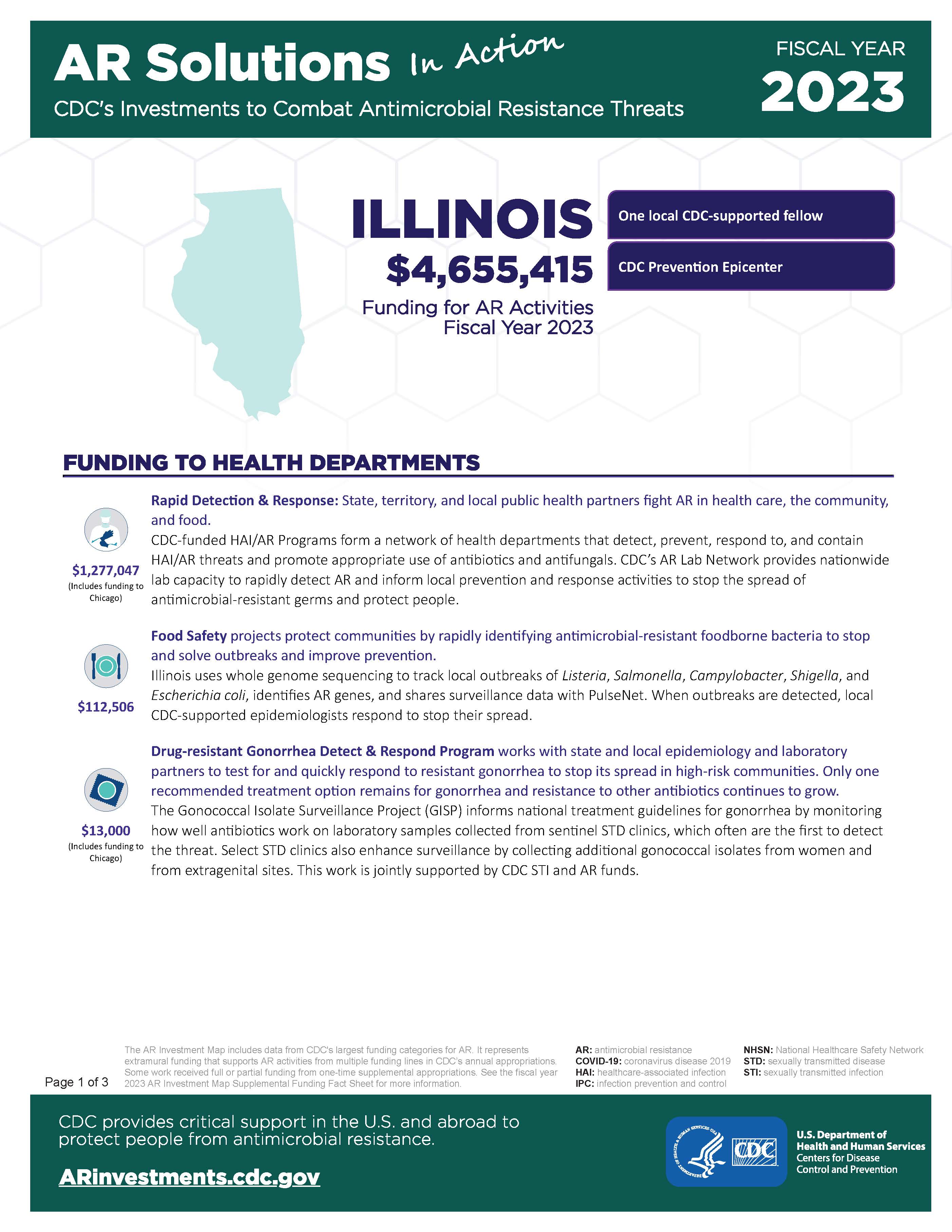The image depicts a detailed infographic titled "AR Solutions in Action, Fiscal Year 2023: CDC's Investments to Combat Antimicrobial Resistance Threats." The primary focus is on the state of Illinois, highlighted with a green outline. Illinois is identified as receiving $4,655,415 in funding for antimicrobial resistance (AR) activities for the fiscal year 2023. Key elements of the graphic include:

1. **Funding Allocation and Programs**:
   - Illinois funding breakdown:
     - $1,277,047 allocated to Chicago.
     - Grants to health departments for rapid detection and response to AR threats.
   - Support for one local CDC-supported fellow.
   - Inclusion of a CDC Prevention Epicenter.
   - Financial support for state, local, and territorial public health partners combatting AR in healthcare, the community, and food.

2. **CDC's HAI/AR Programs**:
   - A network of health departments is funded to detect, prevent, respond to, and contain healthcare-associated infections (HAI) and AR threats.
   - Promotion of the appropriate use of antibiotics and antifungals.

3. **AR Lab Network**:
   - Provides nationwide lab capabilities to rapidly detect AR.
   - Informs local prevention and response activities to halt the spread of AR germs.

4. **Food Safety Projects**:
   - Funded with $112,506 for projects that rapidly identify antimicrobial resistance in foodborne bacteria.
   - Aim to stop and resolve outbreaks and enhance prevention efforts.

5. **Drug-Resistant Gonorrhea Detection and Response Program**:
   - Allocated $13,000 to detect and respond to drug-resistant gonorrhea cases.

6. **Global and National Support**:
   - The CDC provides essential support within the U.S. and globally to safeguard populations from antimicrobial resistance.
   
   At the bottom, the infographic provides a reference to the AR Investments website (ARinvestments.cdc.gov) and features the CDC's blue and white icon.